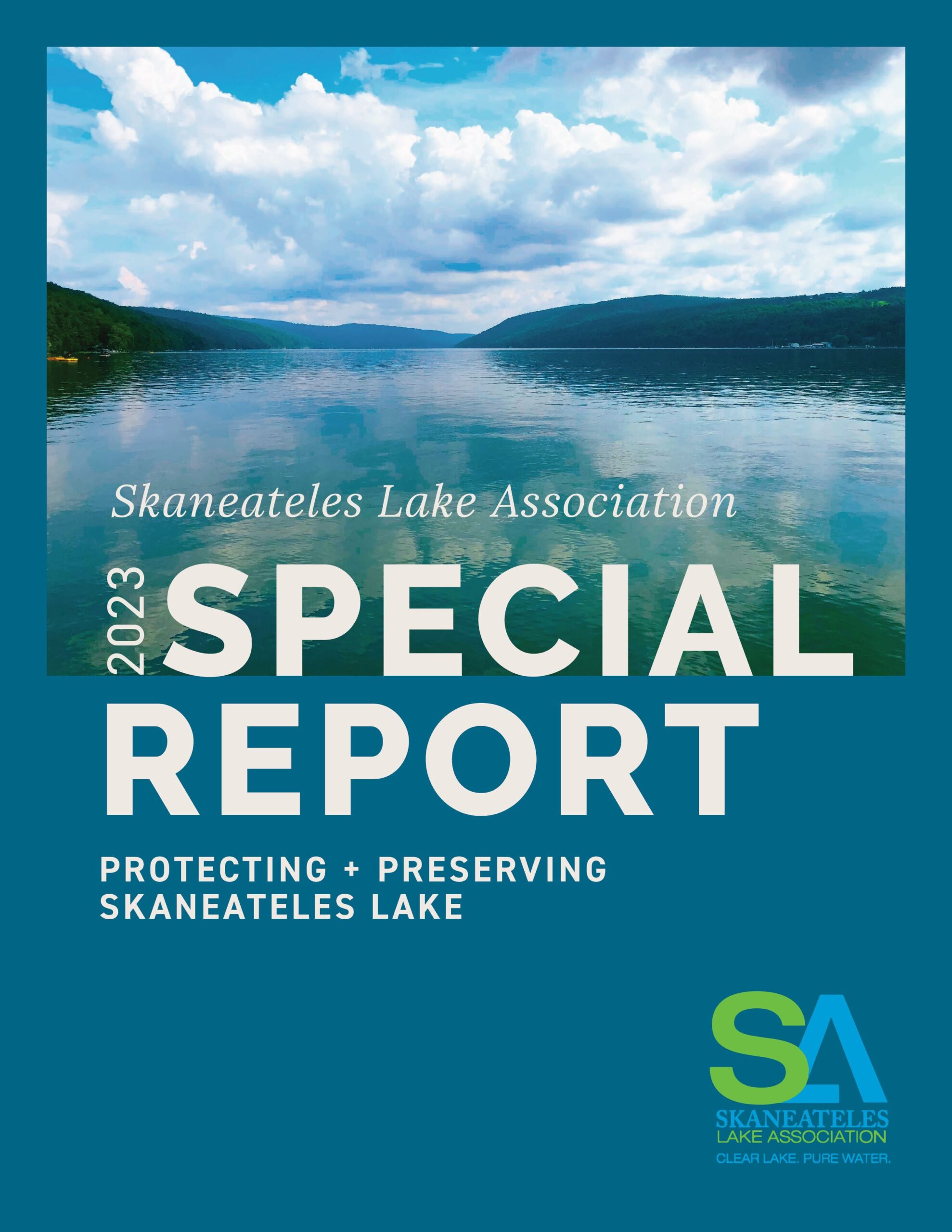This promotional image, likely seen on a poster or website banner, features a striking, serene lake scene with Skaneateles Lake as the centerpiece. The lake is narrow and stretches out long, enclosed by verdant hills that descend toward the calm waters. Puffy white clouds drift in the sky, interspersed with some darker gray ones. Overlaid on this picturesque setting, in bold white text, are the words: "Skaneateles Lake Association 2023 Special Report: Protecting & Preserving Skaneateles Lake." The entire backdrop is set against a navy blue background, enhancing the natural greens and blues of the landscape. In the bottom right corner, the Association’s logo—a green 'S' and a blue 'A'—along with the slogan "Clear Lake, Pure Water," is prominently displayed. This cover page effectively captures the beauty and tranquility of Skaneateles Lake while emphasizing the Association’s commitment to its preservation.